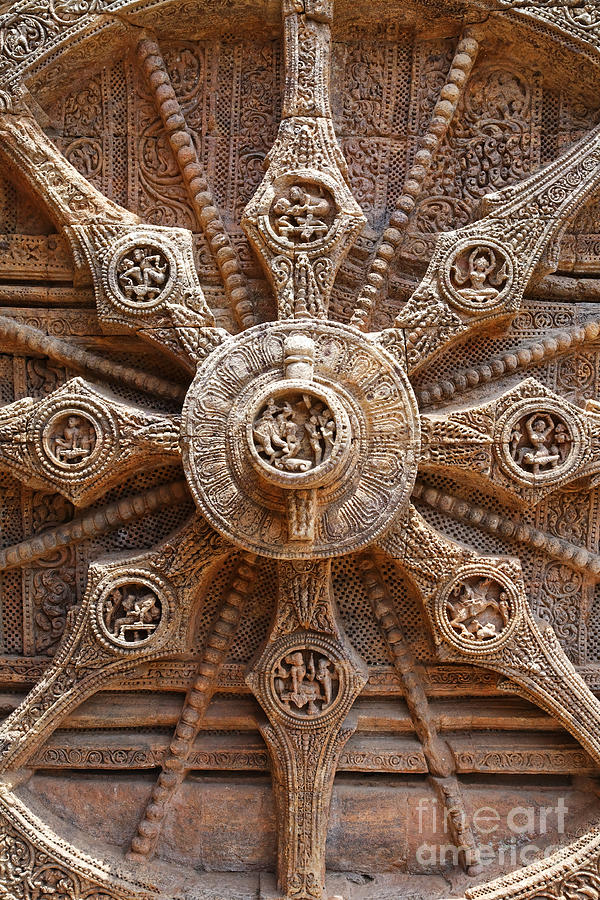The image depicts a highly intricate and ornately carved section of a temple's exterior wall made of brown stone, appearing somewhat similar to a large, circular sculpture. The centerpiece is a circular medallion featuring a detailed engraving of human figures. Radiating from this central circle are eight branching spokes, each adorned with intricate patterns and additional carvings of various subjects, predominantly human figures. Among these carvings, there are depictions of a lady sitting and dancing with both hands raised, touching each other, as well as images resembling horses. The entirety of this ornate structure is rich with fine inscriptions and detailed sculptures. Notably, the bottom right corner of the image is marked with the words "Fine Art America," suggesting the photograph's acknowledgment by the art platform.